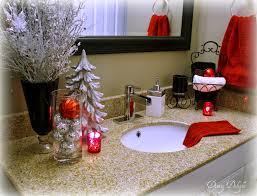This image captures a holiday-themed bathroom countertop, meticulously decorated to evoke the spirit of Christmas. The single white sink features a polished silver faucet, over which a red square cloth—likely a washcloth or cup towel—elegantly drapes, partially dipping into the basin. The speckled countertop, which could either be genuine granite or a high-quality laminate imitation, serves as the foundation for an array of festive decorations.

To the left of the sink stands a distinctive brown pedestal vase, accented with a clear base. The vase is filled with spray-painted white reeds, contributing to the wintry ambiance. Above the countertop, a brown-bordered mirror reflects the scene, adding depth to the small space. On the right wall, a clear-hoop towel rack holds a red towel, matching the overarching holiday color scheme.

Scattered across the countertop are several red votive candles, their warm glow enhancing the festive atmosphere. A small white Christmas tree sits close to the faucet, adorned with additional red votive candles around it, completing the Christmas decor with a touch of elegance and charm.